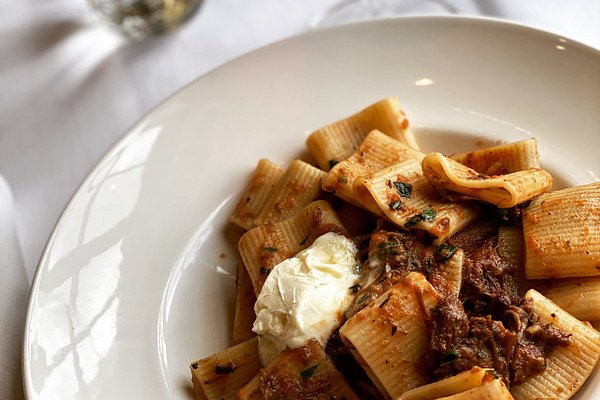This high-definition photograph captures a gourmet dish set against a white tablecloth with noticeable folds, hinting at an elegant dining setting. In the background, partially blurred, are hints of glassware and other dishware, suggesting a prepared table. The central focus is a round, white plate with a deep center, resembling a pasta bowl. It holds rigatoni pasta, generously ridged and sauced lightly with a tomato-based meat or marinara sauce, accented by possible sun-dried tomatoes or small pieces of meat. The dish is garnished with green herbs or spices, likely parsley. On the left side of the rigatoni, there is a small dollop of what appears to be burrata cheese, adding a creamy texture to the presentation. The photograph's lighting captures reflections, possibly from a nearby window, highlighting the textures and colors of the dish, making it appear exceptionally vivid and appetizing.